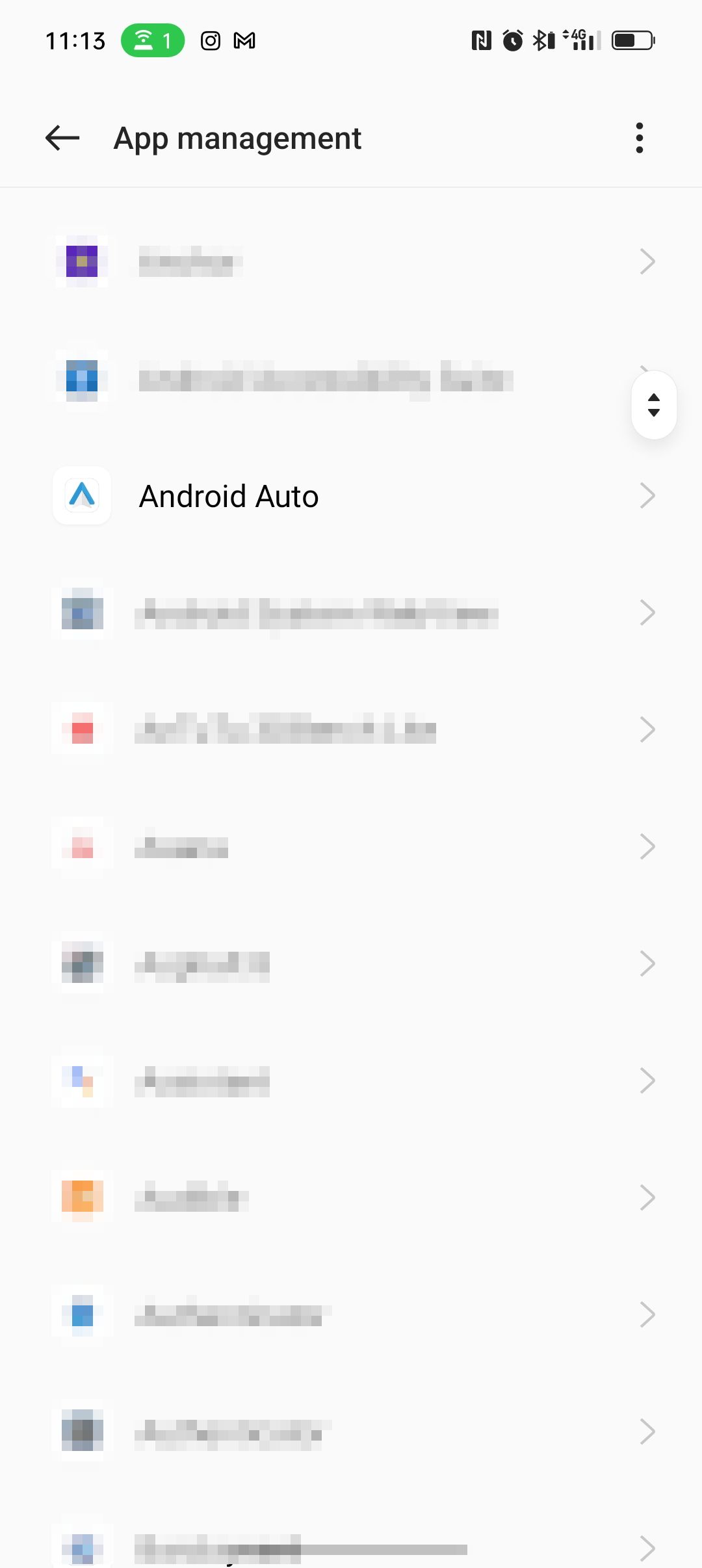Sure, here is a cleaned-up and detailed caption for the image:

---

"A screenshot of a cell phone screen featuring a white background with black text at the top displaying '1113'. Beneath the time, there's a green icon with a white Wi-Fi symbol and the number '1'. The screen also features the Instagram logo and a mail icon in black. On the right-hand side, there are several other icons including a stylized 'N', an alarm clock, and a Bluetooth symbol. It also shows '4G' indicating cellular service, with the battery level at approximately 50%. Below these, on the left side, there's an arrow pointing to the left with text that appears to be 'App Management'. A row of three buttons is visible, followed by multiple gray-out sections. The third item down features a white box with an upside-down blue 'V', and next to it, 'Android Auto' is written in black text on a gray background. On the right-hand side, there's a gray 'greater than' symbol. Above it, a scroll bar is visible with a black up arrow and a black down arrow. The image is otherwise devoid of additional content."

---